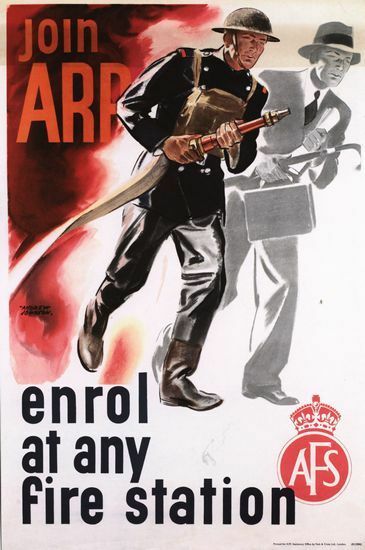This vintage advertisement poster promotes volunteer firefighter recruitment, urging viewers to "Join." Dominating the image is a soldier-like firefighter, clad in a dark World War I-era uniform with silver buttons, a round metal helmet, and big rubber boots. He carries an inactive fire hose and has a pack on his chest. To his right, in a black and white depiction, the same man appears as a businessman in a suit and tie, with a hat featuring a black band, dress shoes, and carrying a briefcase and an umbrella. Red flames blaze on the left side of the poster, adding a sense of urgency. The top of the poster has incomplete orange text, "JOIN AR...", and at the bottom, "enroll" is spelled out in black text. Below that, a red circle with a crown emblem contains the letters "AFS" in white. The caption emphasizes that anyone, even an ordinary businessman, can enlist at "any fire station."